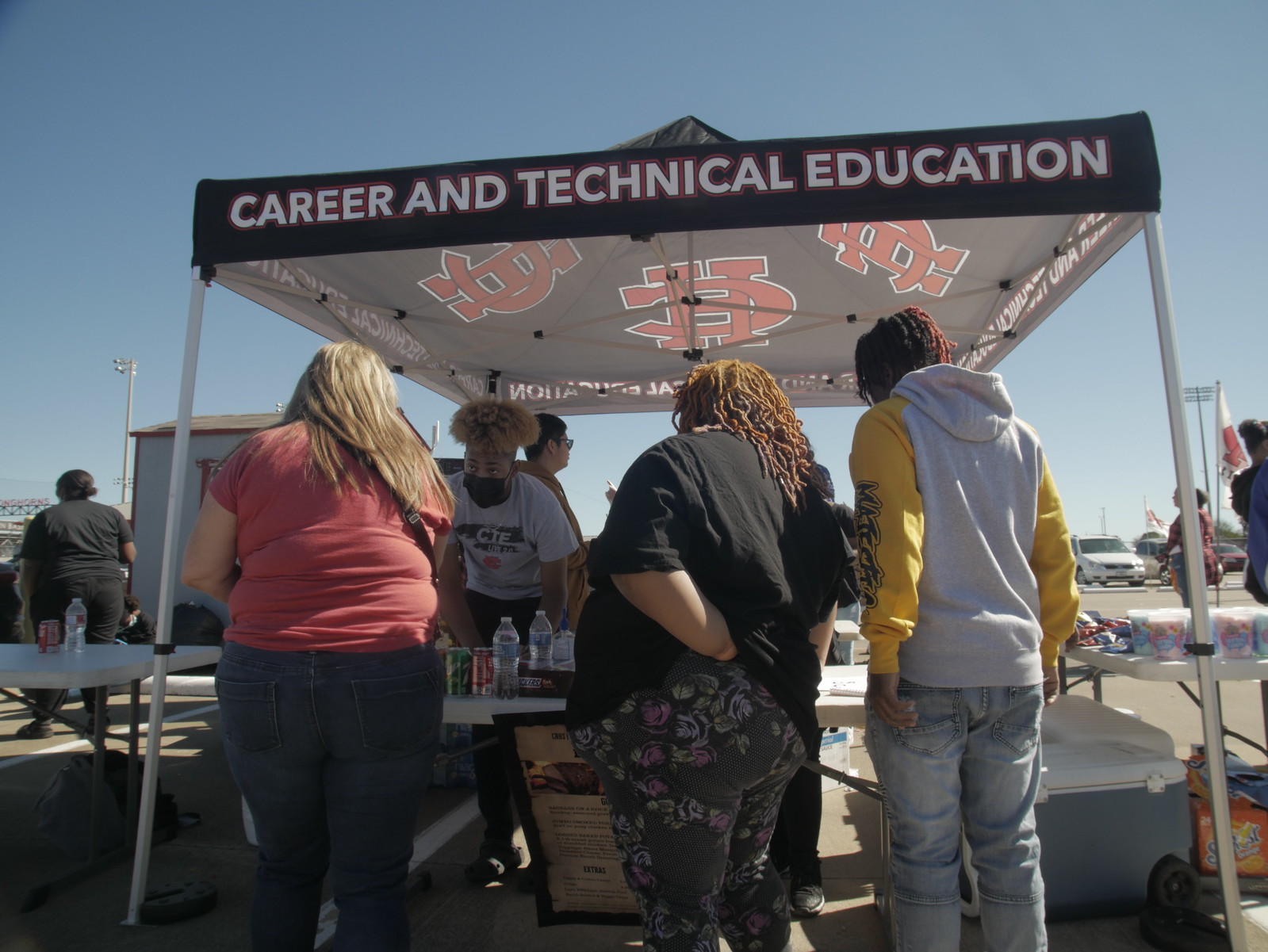In the parking lot of what appears to be a stadium, an open-air job fair is in progress with a prominent black tent featuring white lettering that reads "Career and Technical Education." On top of the tent, there's a university logo, possibly resembling an "HC," though it’s hard to distinguish clearly. Underneath the canvas cover, three people are standing at the informational table. To the side, several helpers provide information about Career and Technical Education (CTE). The front of the booth faces outward to the fairgoers. 

A man with a distinctive golden afro, full dark beard, and dressed in a white T-shirt, blue jeans, and sneakers stands inside the tent. He converses with someone whose hand is only visible. At the table, which doubles as a refreshment stand, a variety of snacks are displayed, including bottles of water, Snickers bars, Sprite, and Coca-Cola, with coolers placed under the right side of the table.

Interacting with the booth are two women and a man. The first woman has blonde hair, is wearing a pink top and wide blue jeans. The second woman sports reddish cornrows, a black T-shirt, and floral-patterned pants. The third person is a young man in a sweatshirt with a white body and yellow sleeves, coupled with blue jeans. Surrounding the booth, a few attendees stand and observe, contributing to the bustling atmosphere of the job fair.